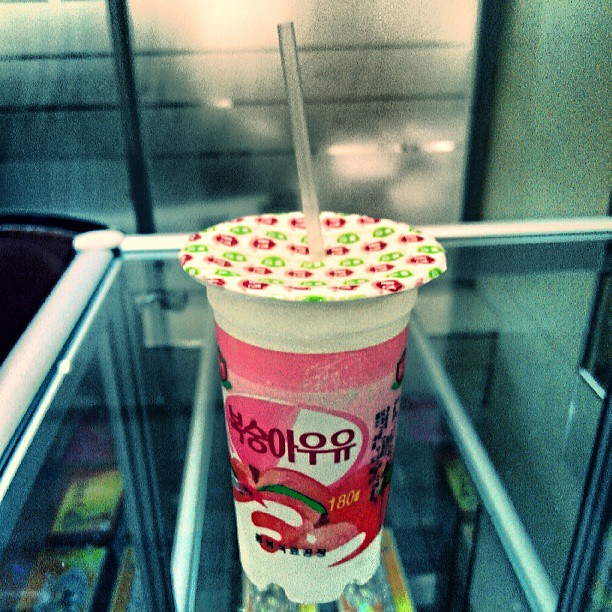This indoor image captures a vibrant, possibly Japanese drink presented prominently in the center. The drink is housed in a white cup adorned with colorful lettering in hues of pink, green, black, and white. A clear straw punctures through a sealed plastic lid for spill-free sipping. The text on the cup, including "180" in bright yellow, seems to feature multiple languages, adding to its exotic appeal. The drink rests atop a glass countertop, beneath which other indiscernible items reside. The backdrop showcases frosted glass windows, white walls, and muted silver and gray tones, creating a clean, minimalistic setting. The overall scene exudes a calm indoor atmosphere, likely within a store or café.